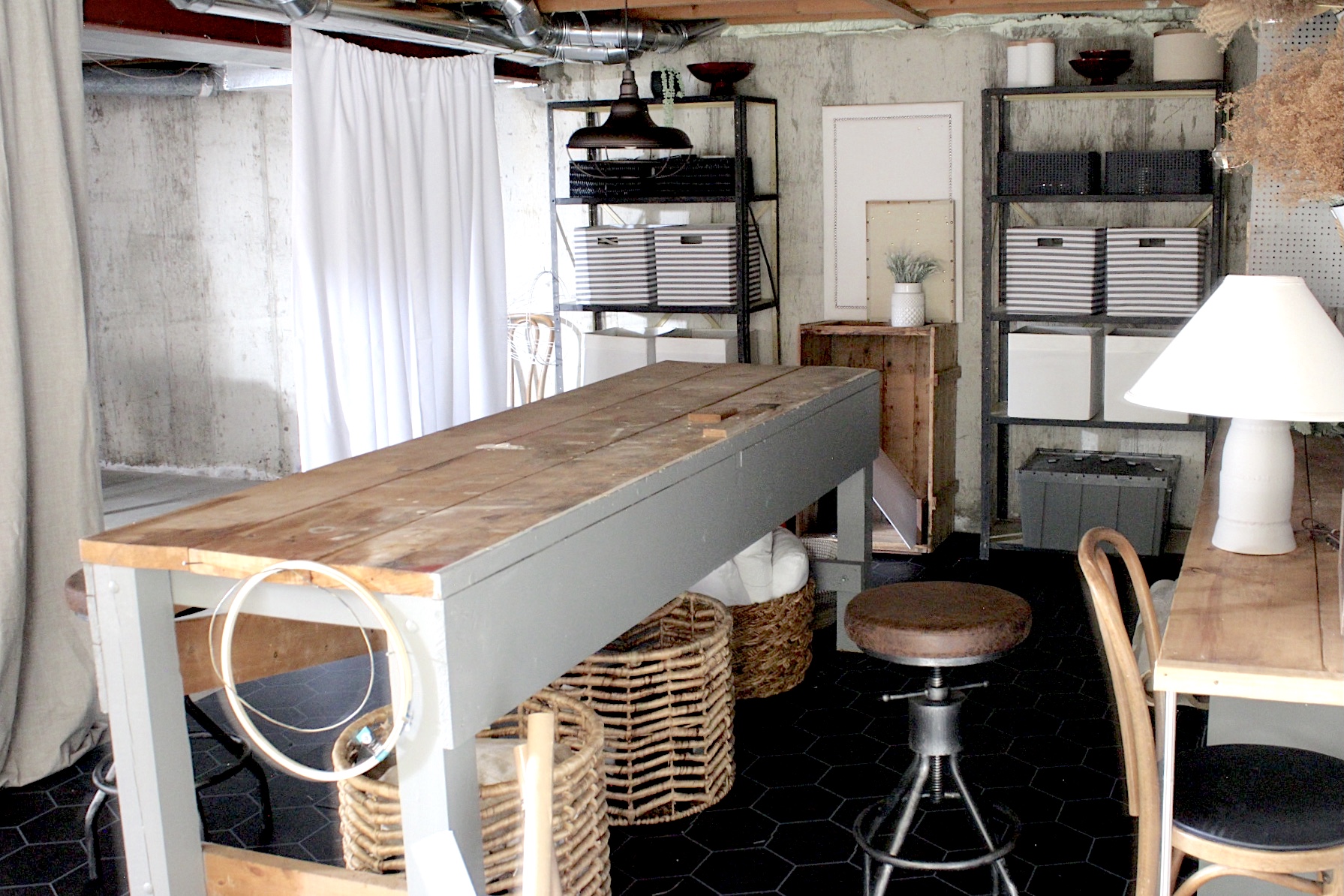This is a detailed photographic image of an indoor workshop area, likely situated in a basement. The central focus is a wooden table composed of three wood planks, painted white around the edges, and supported on the bottom with three large wicker baskets for storage. Behind this table stands a brown-seated metal stool with a screw mechanism to adjust its height. Adjacent to the stool is another wooden table, partially obscured by a tucked-in chair, which features a white ceramic lamp with a white lampshade.

The back of the room showcases industrial-style gray metal shelving units. These shelves contain various storage boxes, including cloth bins with white labels, a bowl, and a vase with green plants. In between the shelving units is an additional bookcase, adding to the room's storage facilities. To the left, a white curtain that can be moved horizontally indicates a partition between the workshop and an open area of the basement, where concrete walls and floors, along with HVAC equipment, are visible. 

The floor under the work area consists of hexagonal black tiles with white mortar lines, enhancing the industrial aesthetic of the space. The precise organization and design elements, including dried plants in the top right corner, contribute to a functional and aesthetically pleasing workshop environment.